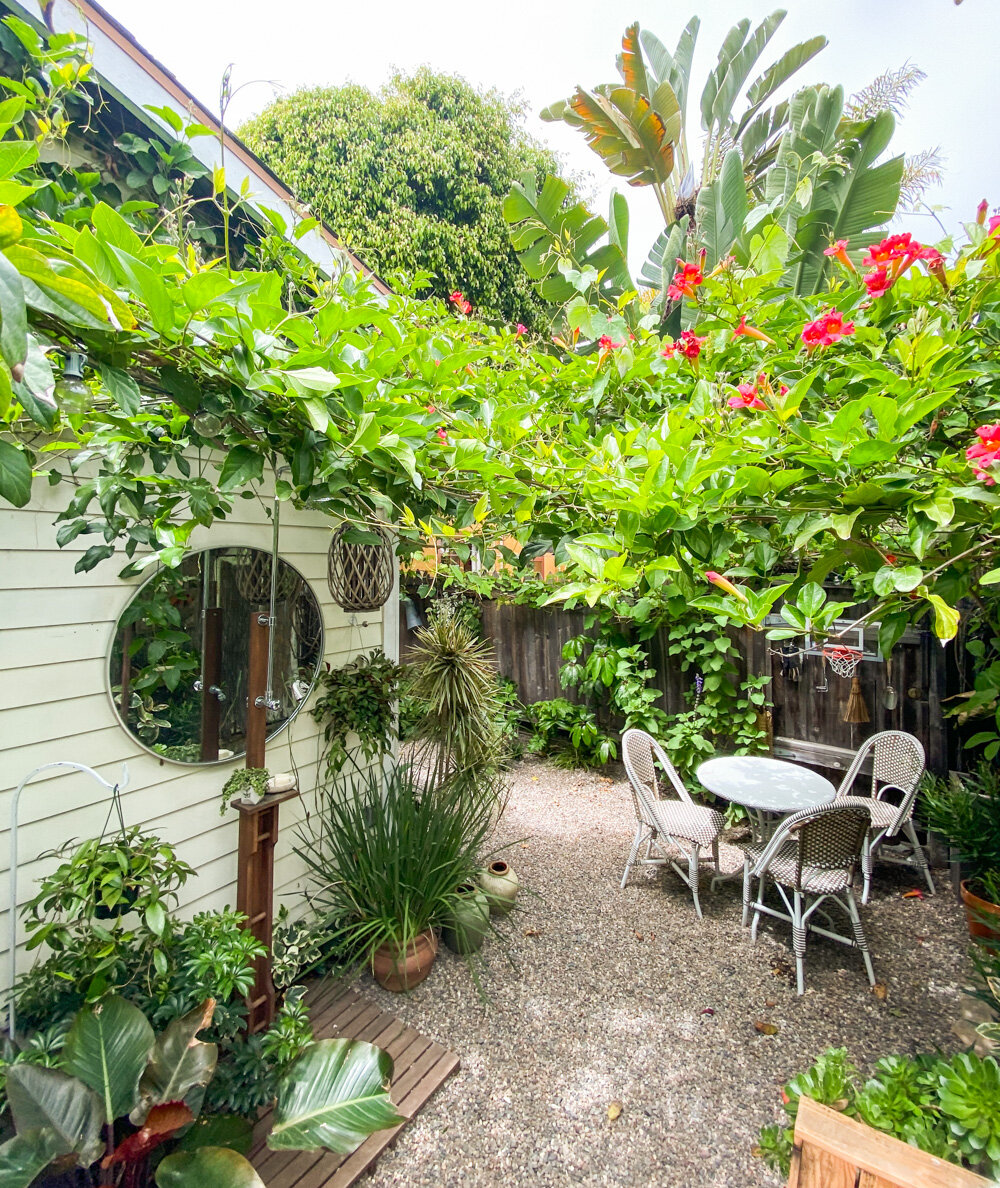The photograph captures an outdoor scene set in what appears to be a charming and vibrant backyard garden during daytime. The left side of the image features a house or shed with white siding, adorned with a round mirror mounted on the wall. In front of this wall is a collection of potted plants, adding lush greenery to the scene. 

Suspended from the roof of the shed to a fence on the right are hanging green plants, creating a canopy-like effect. A brown metal tower stands prominently on a wooden stand among the plants, while a white stand in the lower left corner supports more hanging plants. 

Diagonally across from the shed, in the top right corner, a cozy seating area is visible. This area includes an oval-shaped metal table surrounded by three outdoor chairs, arranged in a corner formed by a gray fence. Behind the chairs and interspersed among trees, a small basketball hoop is partially obscured by foliage. Further into the background, large-leaved banana plants and vibrant red flowers, resembling trumpet lilies, add bursts of color and height to the garden. The ground is mostly gravel, and scattered ceramic planters contribute to the overall lush, green ambiance.